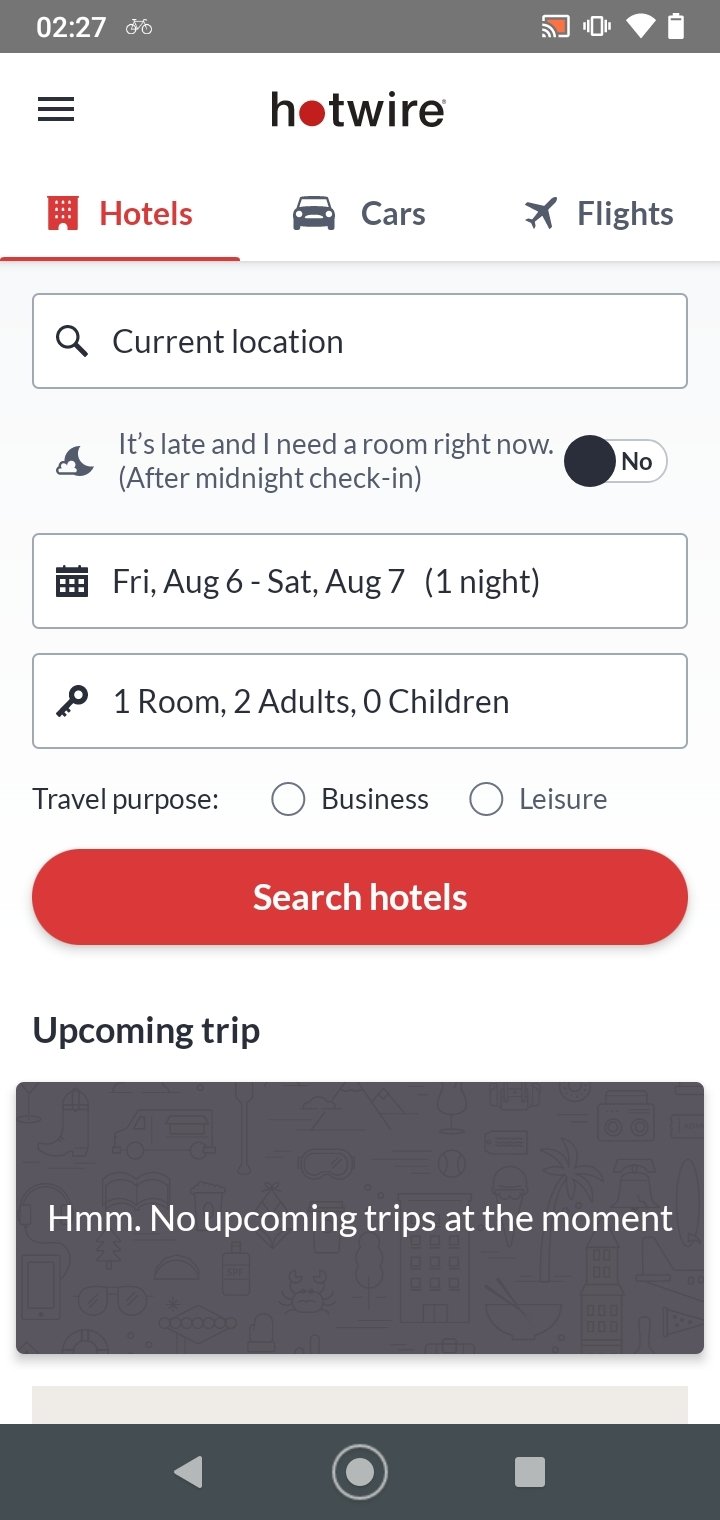This is a detailed descriptive caption for the given image:

---

The screenshot displays the HotWire application on a cell phone. The status bar at the top shows it is 2:27, with icons indicating eyewear (possibly eyeglasses) or a bicycle, and that the device is casting/sharing its screen. Additionally, the status bar shows vibrations are on, Wi-Fi is full, and the battery is nearly full. Below the status bar, the background transitions to white and prominently features the HotWire logo centered at the top. 

To the left of the logo is a hamburger menu icon. Beneath the logo are three large, selectable icons representing "Hotels," "Cars," and "Flights," each accompanied by corresponding graphics of a hotel, car, and airplane. The "Hotels" option is selected, highlighted in red, whereas the other options remain black.

The background then shifts to gray. The first feature is a search bar for the current location. Beneath it, a message states, "It's late, and I need a room right now (after midnight check-in)," with a slider option next to it. Below this is a calendar icon on the left side of a date block displaying "Friday, August 6th, through Saturday, August 7th, one night." The next section features a key icon with text indicating "one room, two adults, zero children."

Further down, a section labeled "travel purpose" offers choices between business and leisure. A prominent red oval button below this text reads "Search Hotels" in white. Subsequent text in bold states "Upcoming Trip," followed by a dark gray block indicating "No upcoming trips at the moment." The screen concludes with a short white space and a gray bar, then the standard black navigation bar at the bottom of the phone, featuring a triangle, a circle within a circle, and a square.

---